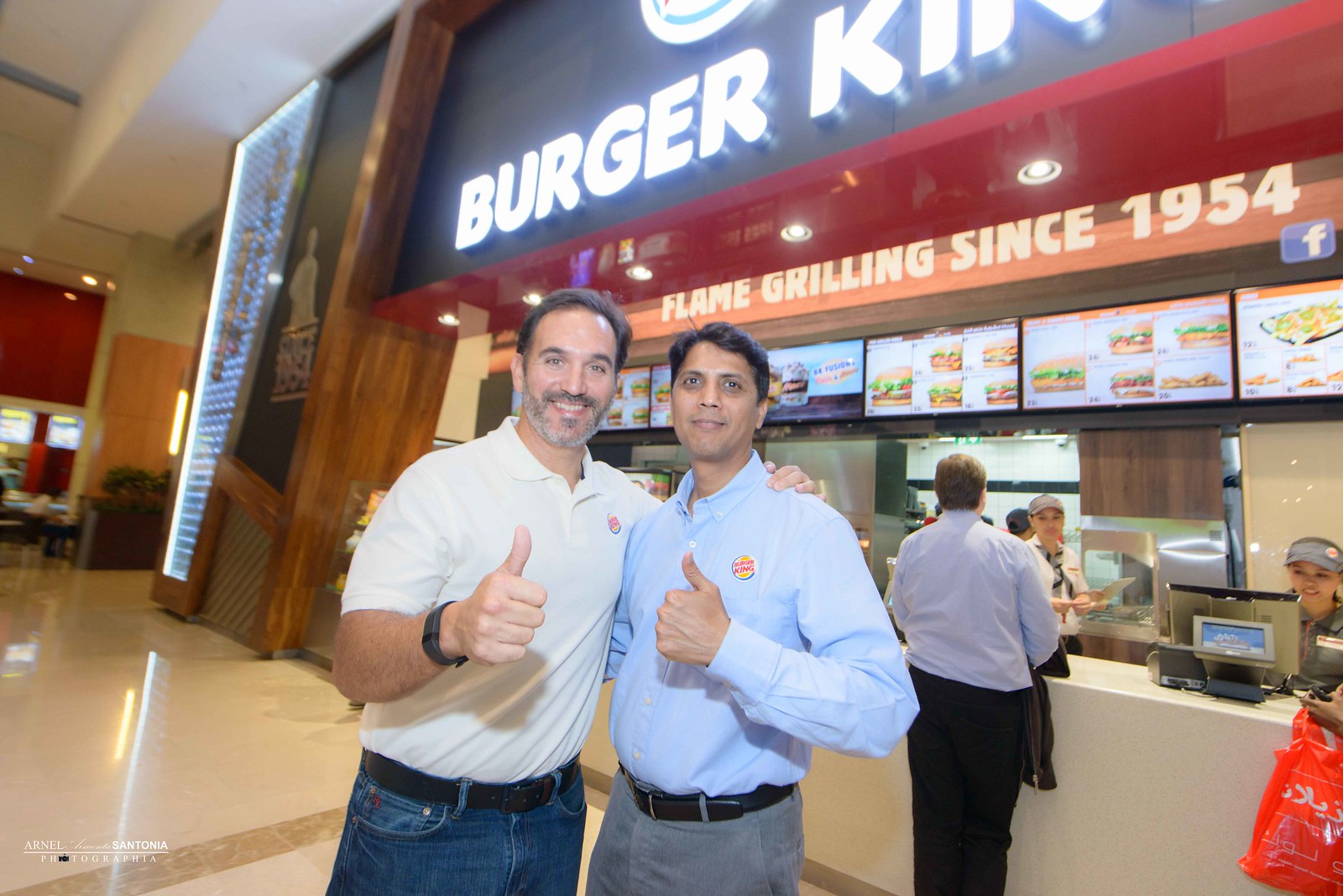The rectangular photograph captures an indoor setting, likely a mall or a roadside stop. Dominating the foreground are two smiling gentlemen standing in front of a Burger King counter. The man on the left, with tanned skin and black hair, is dressed in a white pullover shirt, blue jeans, and a black belt. He has his right arm around his companion and is making a thumbs-up gesture. The man on the right sports a grey beard and moustache, and he wears a blue button-up collared shirt with the Burger King logo and grey trousers, also completing the thumbs-up pose. Both men give a sense of camaraderie as they pose together.

Behind them, the Burger King counter features a large blue sign with glowing lights displaying "Burger King" and the slogan "Flame Grilling Since 1954" on a bright orange banner. The background reveals the bustling interior of the fast-food restaurant, complete with menu boards, order screens, and employees in action. One worker on the far right is taking an order at the checkout, while another assists a customer at the counter. The ambiance and the interaction of both men and staff suggest a warm and lively atmosphere.